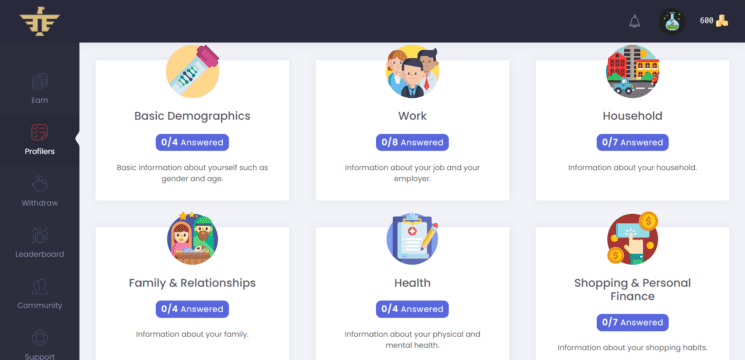The image depicts a profile page layout from Prolific's website. The interface is framed by a black horizontal bar at the top and a black vertical bar on the left. The page prominently features the word "Profile" in white, next to a red profile icon. Multiple sections are displayed, each representing different categories that participants need to complete.

The categories and their respective statuses are listed as follows:
1. Basic Demographics - 0 out of 4 answered, with a colorful round image above.
2. Work - 0 out of 8 answered, also with a colorful round image at the top.
3. Household - 0 out of 7 answered, depicted with a cityscape image.
4. Family Relationships - 0 out of 4 answered, highlighted in purple.
5. Health - 0 out of 4 answered, shown with a clipboard and pencil icon.
6. Shopping and Personal Finance - 0 out of 7 answered, illustrated with an online shopping scene, including a hand on a keyboard.

Each section has vibrant and quirky icons, adding a visually appealing and friendly touch to the page. The header includes a profile picture placeholder and a gold icon resembling an upside-down triangle with black details to the left side. The overall page design emphasizes the need for participants to complete their profiles by answering the listed questions.